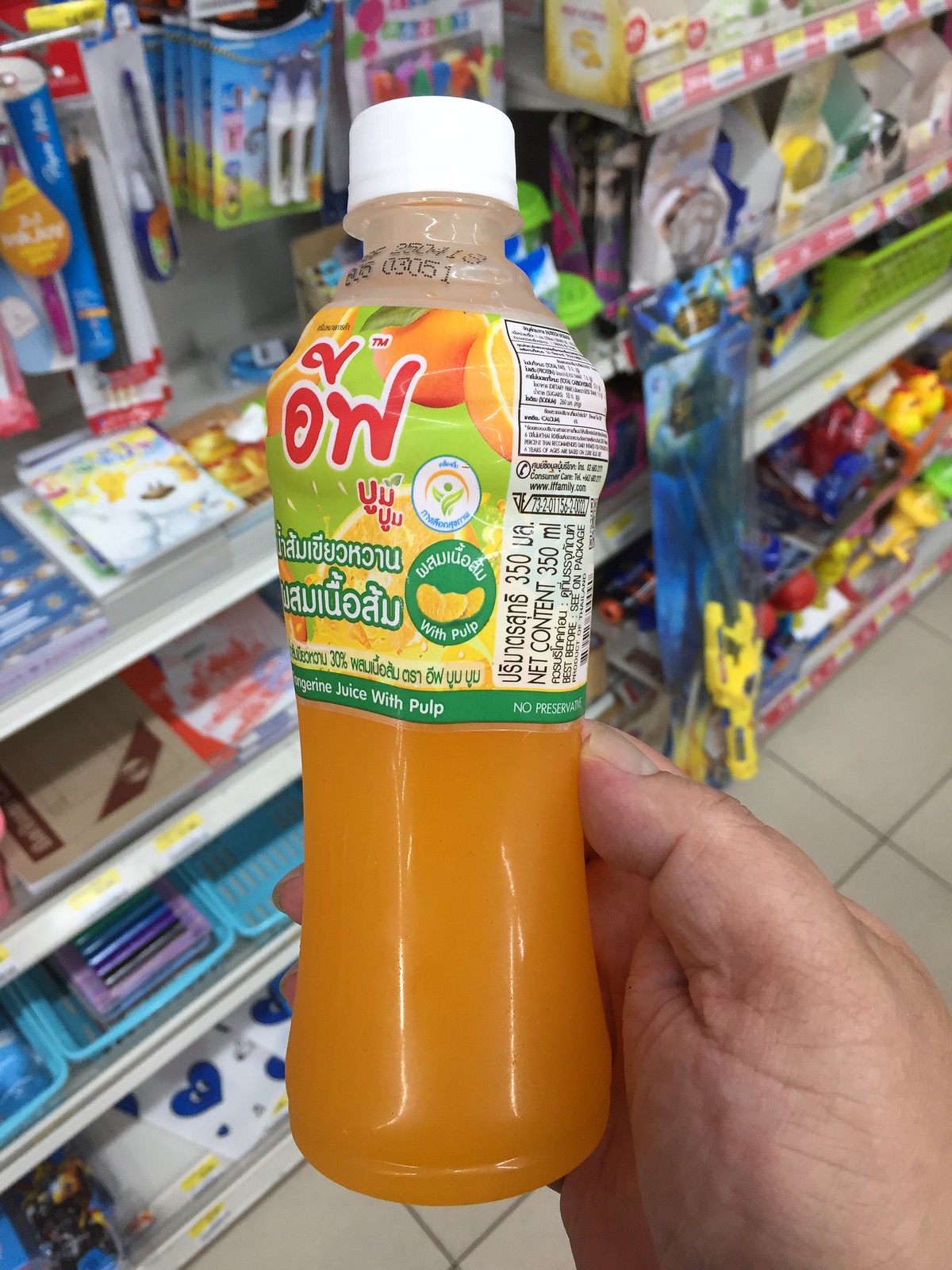This is a color photograph showcasing a close-up view of a drink bottle held by a person's hand. Positioned in the lower right-hand corner, the hand has medium-toned skin, with the wrist securely wrapped around the bottle and the edge of one finger visible. The bottle contains an orange liquid and is capped with a white top. Below the cap, there is some black writing, possibly indicating best-before dates, though it is not legible. The bottle features a vibrant logo adorned with depictions of orange and yellow fruit set against a green background. The logo includes red text outlined in white and white text outlined in green. At the bottom of the label, there is a green rim with additional white text. A nutritional label is partially visible towards the back of the bottle. The scene is set against a grey tiled floor, and in the background, there are shelves stocked with stationery items including pens, pencils, and copybooks, suggesting a retail setting.